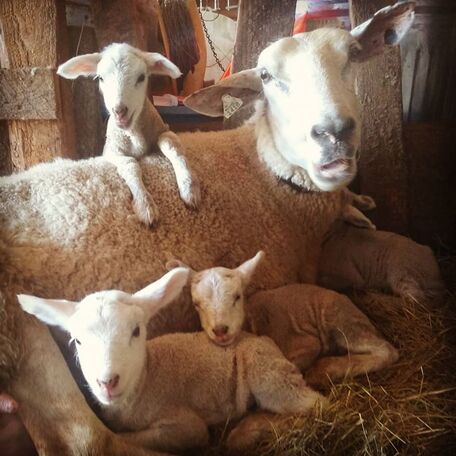In the image, a mother sheep is positioned prominently to the right, her body facing right but her head turned back to look at the viewer with a curious expression. Nestled closely against her are three lambs, each with their tan-colored bodies and white faces. Two of the lambs are pressed snugly against her side, their bodies facing left, while the third lamb has its head hidden under the mother's chest, making it difficult to see its face. Adjacent to these three, the fourth lamb is draped over the mother's back, his body also a blend of tan and white fur. Behind this intimate family grouping, the scene is set inside a rustic barn with wooden beams visible and a floor scattered with straw, adding to the warmth and coziness of the image.